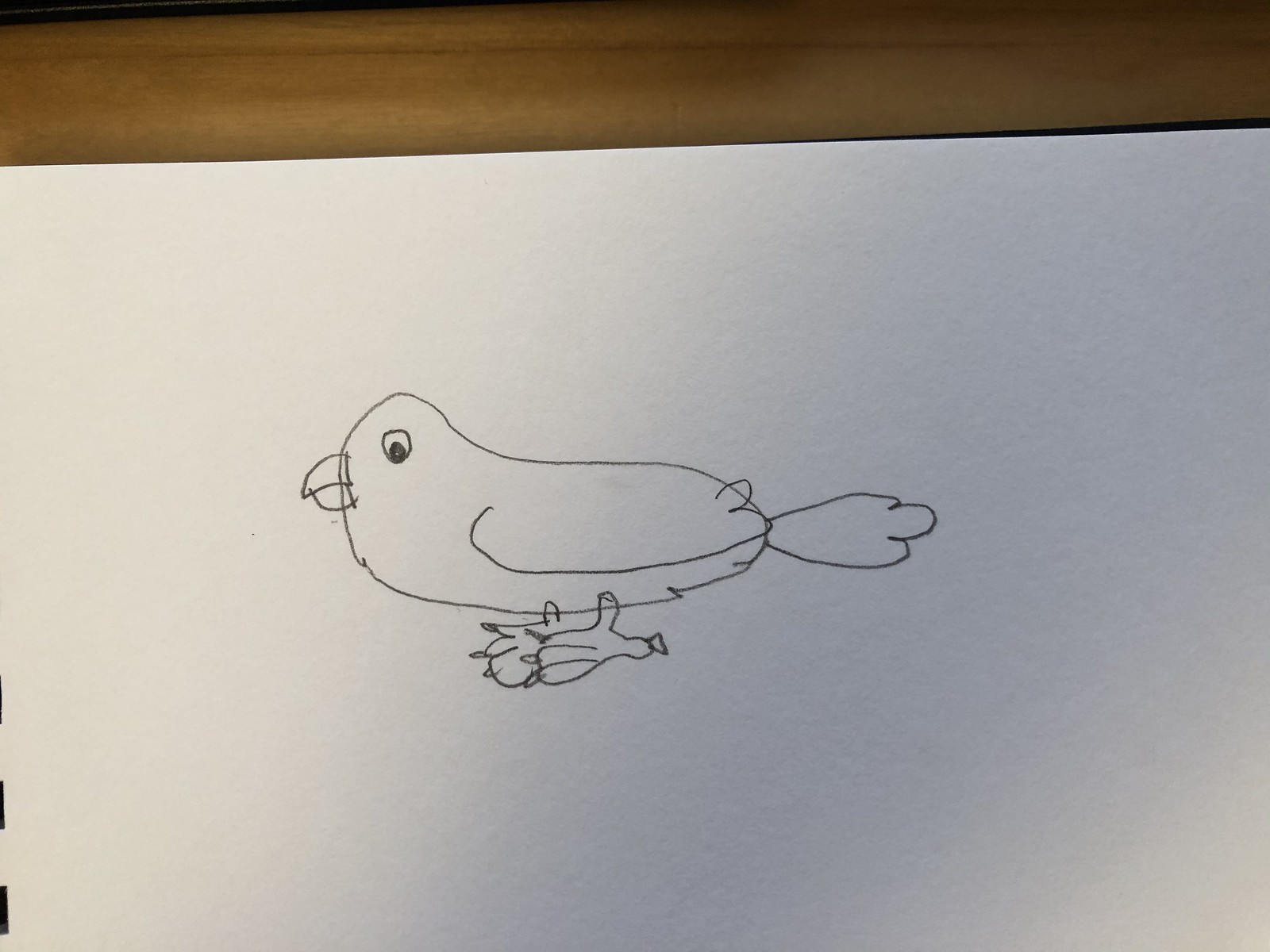A light orchid-colored piece of paper nearly covers the surface of a brown table, leaving a few inches of the tabletop visible at the top. On the paper, a detailed pencil sketch of a small bird is rendered. The bird features noticeably large feet, complete with tiny claws visible at the tips. One of its small wings is drawn with two rounded tips. The bird's tail feathers are prominent, each ending in a rounded tip, and its head narrows to a gentle point. The sketch also highlights the bird's large eye and a petite beak, capturing its delicate features with charming simplicity.